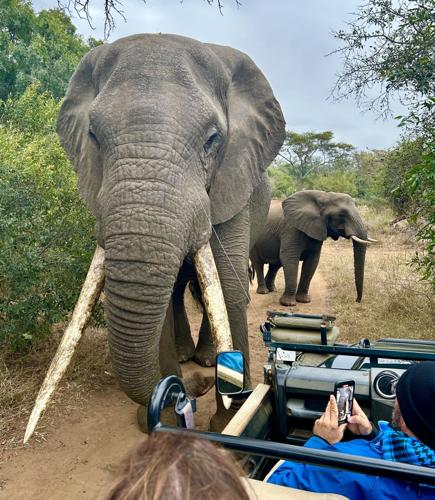The photograph captures a dramatic scene on a dirt path in the wild, likely part of a safari expedition. Dominating the foreground is a massive bull elephant, its imposing stature complemented by exceptionally long, white tusks streaked with brown dirt. This formidable creature is merely steps away from an open-top safari vehicle, intensifying the sense of danger and excitement. The vehicle itself is peopled by a man in a blue jacket, black knit cap, and a blue and black scarf, who is intently snapping photos with his smartphone. In the back seat, another person can be seen, characterized by their brown hair. Surrounding this tense tableau are trees and green bushes, indicative of a biome rich with wildlife. Just behind the bull elephant stands a smaller female elephant with shorter tusks, creating a layered depth to the image. The smaller elephant's large ear and lowered trunk are visible. The expansive background teems with verdant flora, making the scene both picturesque and perilous.